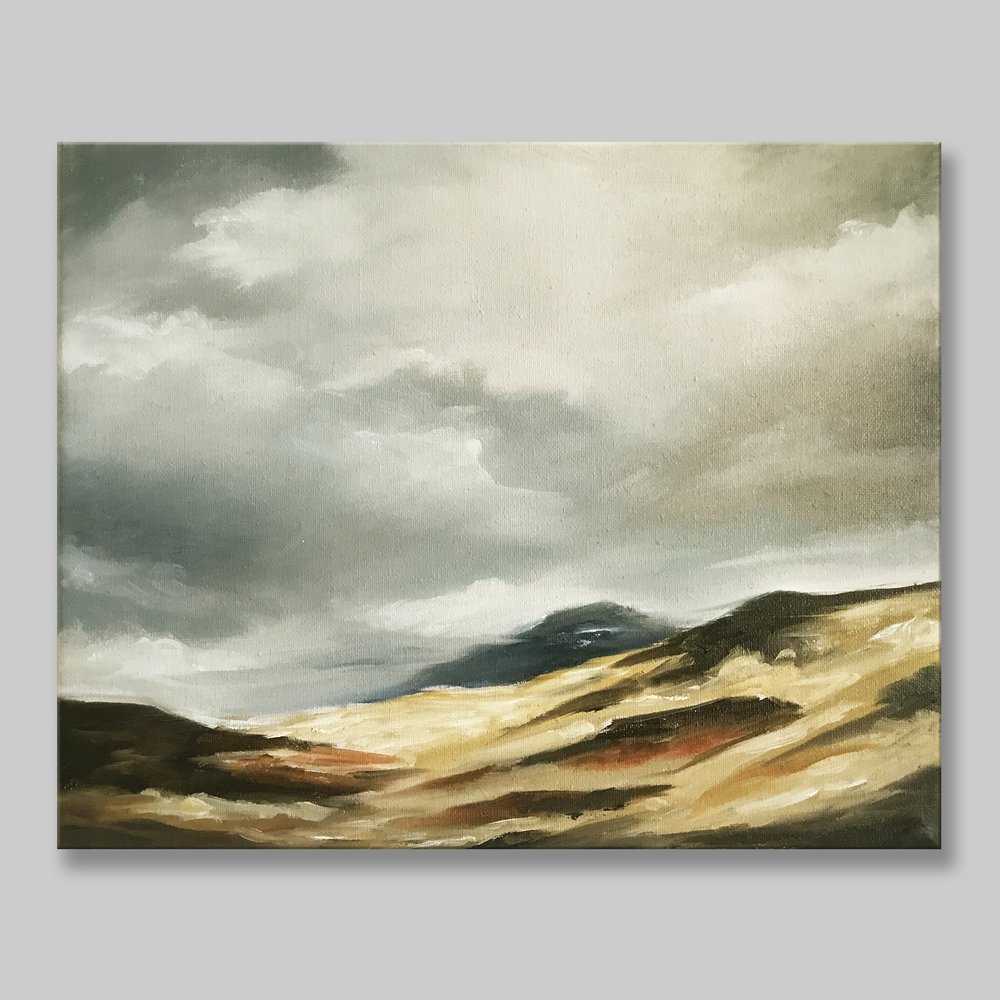The image features a striking painting mounted on a plain, gray wall, casting a shadow that subtly enhances its presence. The wall appears deliberately unadorned, perhaps digitally rendered to emphasize the painting. The artwork itself is square and portrays a dramatic landscape, blending elements of realism and abstraction.

The upper portion of the painting is dominated by an ominous, storm-filled sky, thick with layers of gray and dark clouds but interspersed with lighter areas. These clouds almost seem tangible, their texture rich and brooding, evoking a sense of impending weather.

The lower portion depicts a series of rolling hills, varying in color from light brown and beige to dark brown and nearly black. These slopes dip and rise, with the right side climbing upward into a hill and the left side featuring a predominantly black slope accented with shades of brown. Beyond these hills, there is a grayish expanse that evokes the ocean, adding to the overall stormy and eerie atmosphere of the scene.

Intriguingly, the painting features abstract elements as well, with white strokes suggesting mist, fog, or clouds drifting among the hills, heightening the sense of mystery and surrealism. The combination of detailed, dramatic natural elements and abstract strokes invites the viewer into a turbulent, almost otherworldly landscape reminiscent of a stormy coastal area.